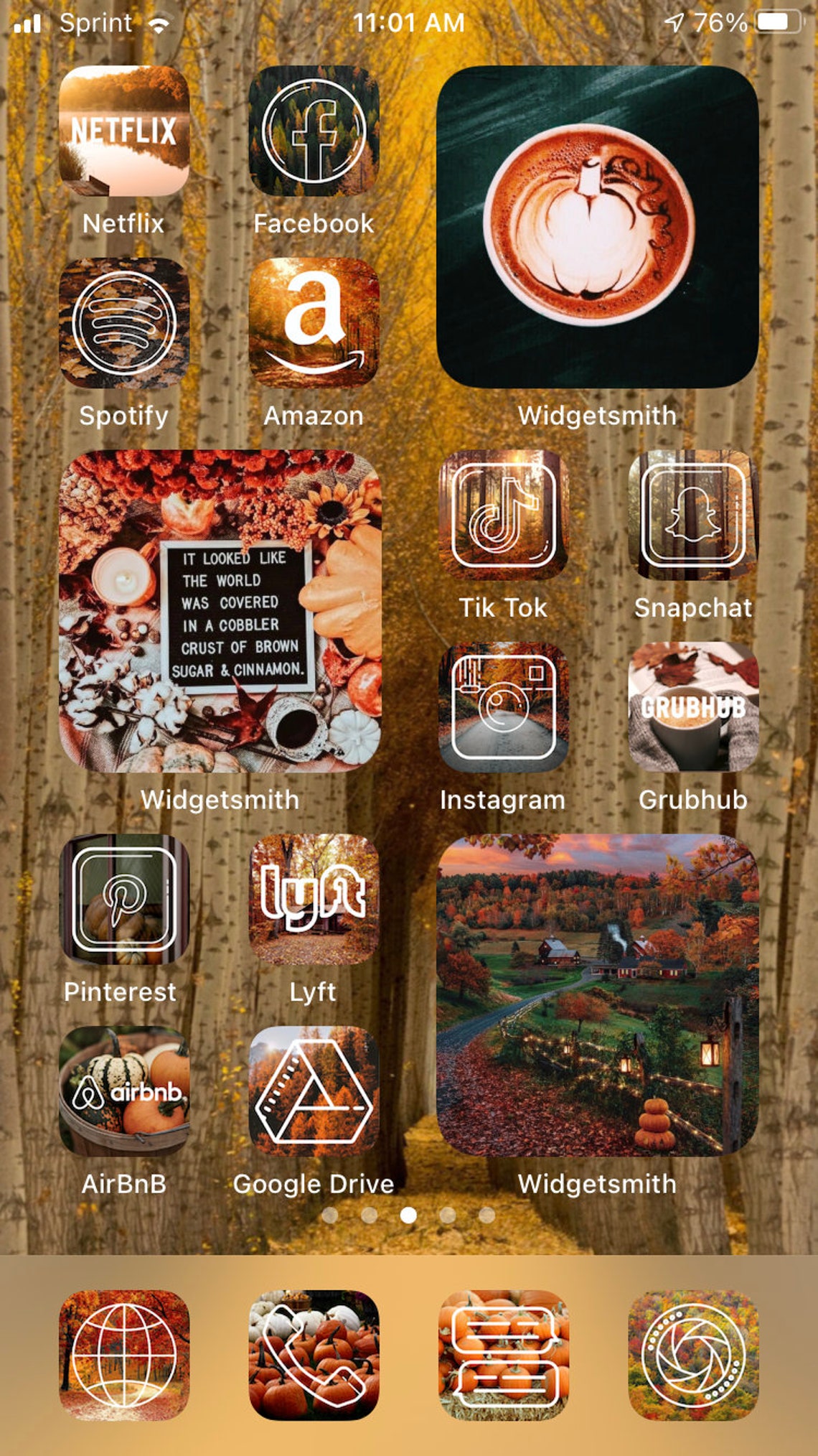The image shows the home screen of a Mac tablet or phone, featuring a vibrant, forestry-themed background. The scene depicts a serene pathway blanketed with golden-yellow leaves, surrounded by light brown trees. The sky above mirrors the color palette with an orange-yellow hue, creating a warm, sandy-toned atmosphere.

At the top left corner, the screen displays the service provider "Sprint," the time "11:01 am," and a battery percentage of "76%". The application icons are designed primarily in white, playing off the sandy theme of the background. The apps visible on the screen include Netflix, Facebook, Spotify, Amazon, and multiple instances of Widget Smith. Additional apps listed are TikTok, Snapchat, Instagram, Grubhub, Pinterest, Lyft, and Airbnb, along with Google Drive.

At the bottom of the screen, four essential icons are neatly arranged: a globe icon presumably for web browsing, a phone icon, an icon with two speech bubbles representing messaging, and a camera lens icon, likely for the camera app.